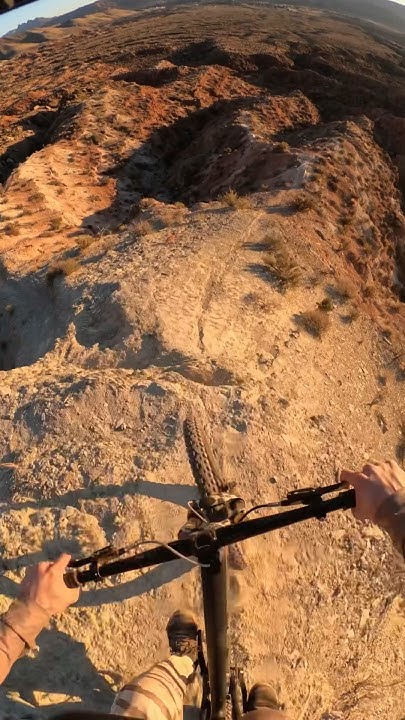This image captures a first-person perspective from someone's GoPro camera, positioned at the top of a narrow, rocky hillside. The view angles downwards, showing the front end of a mountain bike with a dirty front wheel rolling over the rugged terrain. The rider, clad in beige pants with brown horizontal stripes and brown tennis shoes, grips the black handlebars tightly with both hands. Their long-sleeved, brownish shirt contrasts against the light-colored, clay-red dirt and rocks that dominate the scene. The landscape beneath the rider is barren with little vegetation, transitioning from the immediate rocky trail to distant ridgelines and scattered dirt patches. The entire scene is framed against a backdrop of beige and red hues, emphasizing the stark, rugged beauty of the rocky terrain.